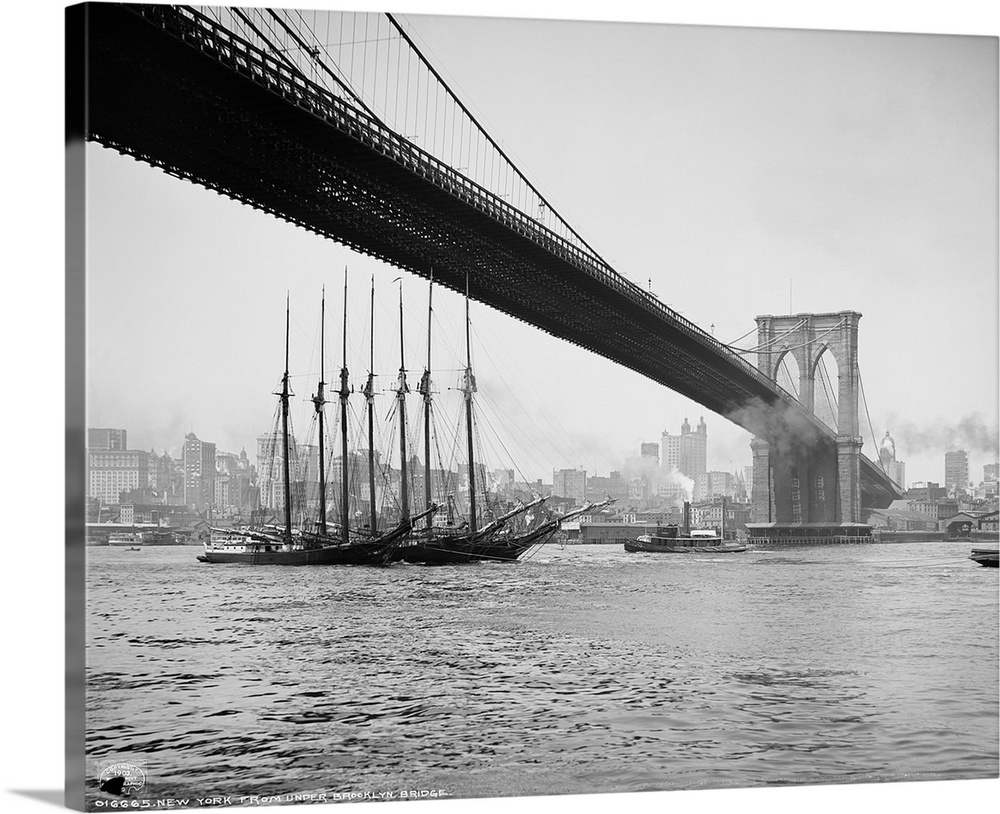This is a black-and-white photograph dating to the late 1800s or early 1900s, depicting the iconic Brooklyn Bridge in New York. The image captures the bridge from the perspective of someone looking up from the water below, with the left side of the bridge extending to the right. The majestic bridge stretches from the top left-hand corner of the image and narrows as it reaches the mid-right, offering a dramatic view of its suspension structure. In the background, the emerging Manhattan skyline is visible, shrouded in smoke and smog typical of the industrial era. 

Underneath the bridge, a slim and streamlined ship with seven masts sails gracefully, hinting at its design for speed rather than cargo transport. Additionally, there is a tugboat navigating near one of the bridge's supports and a ferry in the distant background. Linen boats and parts of the pier are visible near the bridge's arch. The bottom of the photograph bears the inscription in white letters: "New York from under Brooklyn Bridge."